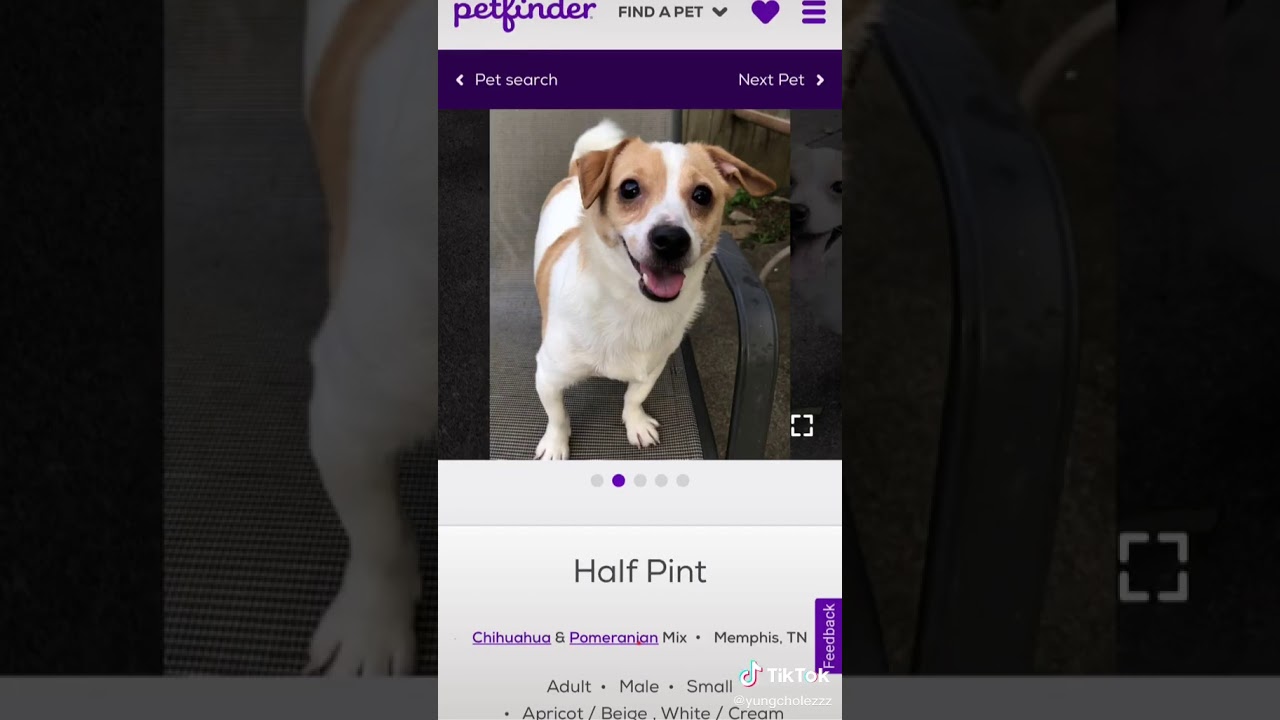Screenshot of a Petfinder webpage featuring a Chihuahua and Pomeranian mix dog named HalfPint. The Petfinder logo appears in the upper left corner in purple cursive font. The webpage includes black text options such as "Find a pet" and "Menu," along with a "Likes" feature in the context menu. HalfPint, described as an adult male with small size, has apricot and beige fur with white and green highlights. The purple text at the bottom confirms the breed as Chihuahua and Pomeranian mix. The dog is located in Memphis, Tennessee. There are options to maximize the image and swipe through pictures at the bottom right-hand side, accompanied by a feed button. The image also contains a faded TikTok watermark in the bottom right corner, suggesting it was first viewed on a computer before being screenshotted on a phone.